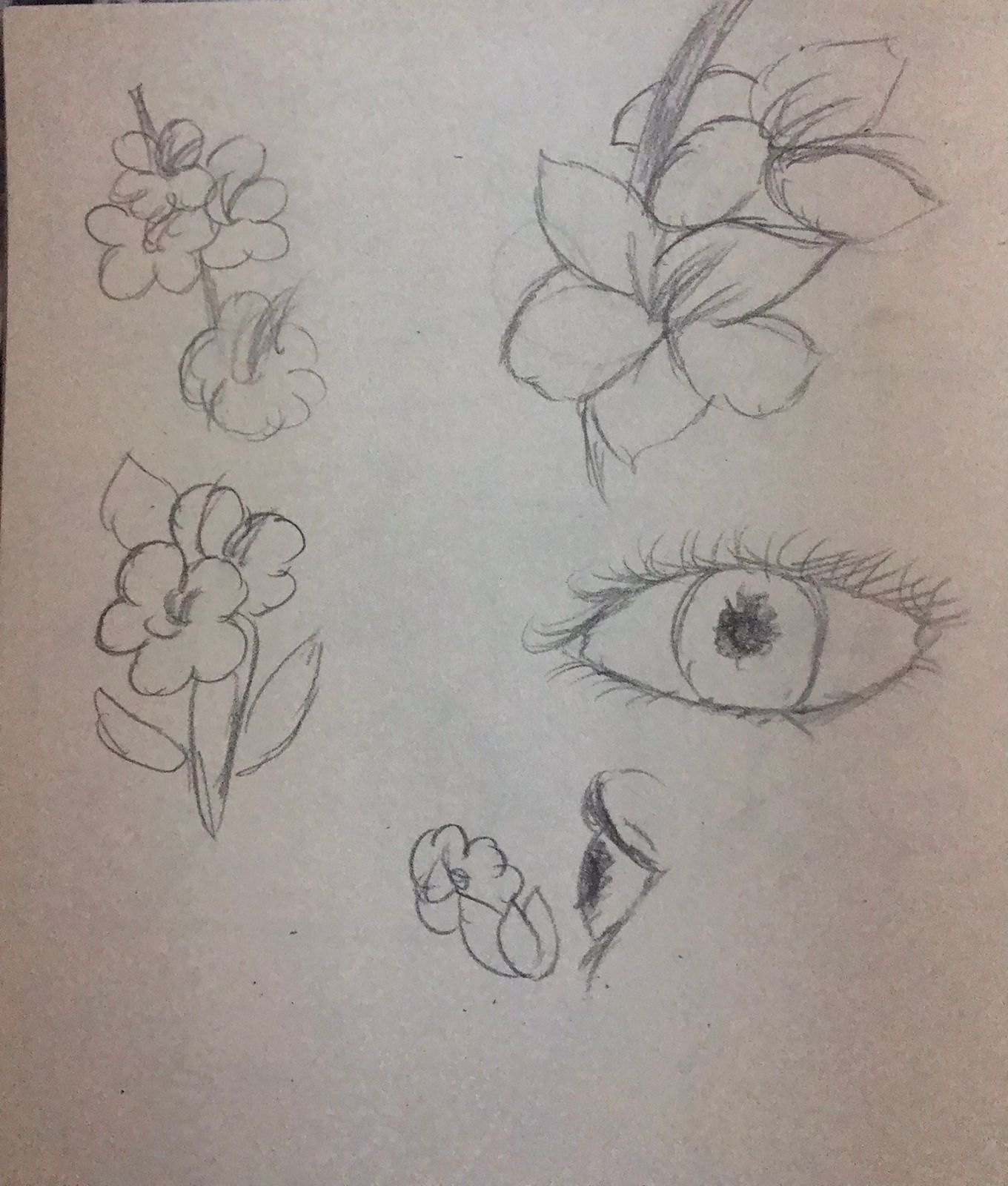This image showcases a single sheet of white paper filled with several pencil sketches. Among the five distinct drawings, three depict flowers with five petals, some stems, and a few leaves. The flowers vary in perspective: one presents a top-down view, while the others seem to float or stand upright. The artist, likely a beginner, has also included two depictions of eyes—one facing forward, displaying detailed eyelashes and a visible pupil and cornea, and another in a side profile appearing to gaze directly at one of the flowers. The drawing features uniform graphite shading with no additional colors. Evidence of erased and redrawn petals hints at the artist's attempts to refine their work.